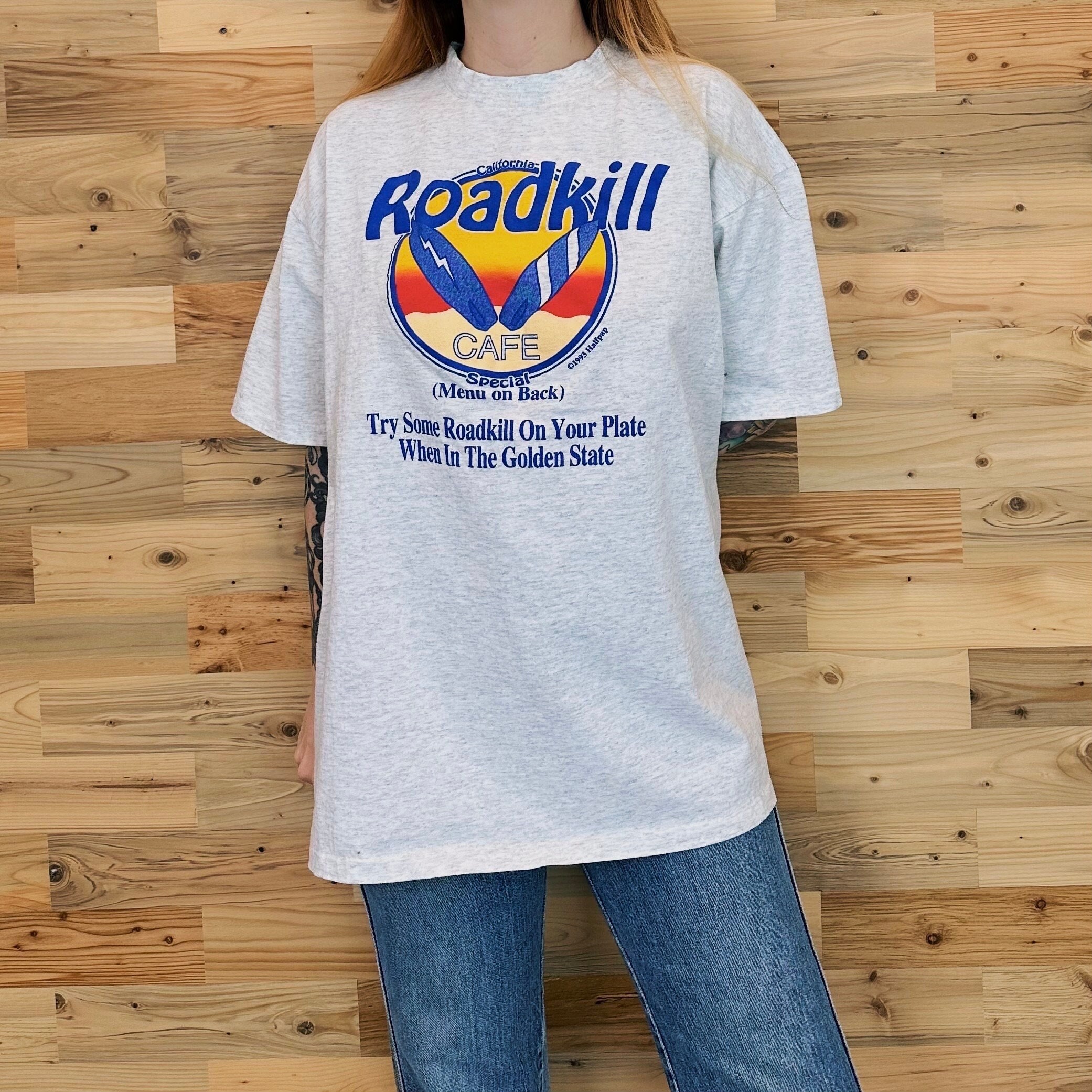In this image, a woman with dirty blonde, shoulder-length hair is modeling a gray heather crewneck t-shirt with short sleeves in front of a knotty pine, woodgrain background. She is wearing blue jeans and has tattoos visible on her right arm and left elbow. The t-shirt features a circular graphic with surfboards propped up on a beach, set against a yellow and red sunset background. The text "Roadkill Cafe" is written in blue within the circle, with "Special Menu on back" and "Try some Roadkill on your plate when in the Golden State" also in blue lettering beneath the graphic. This scene showcases the Roadkill Cafe t-shirt from California in detailed clarity.